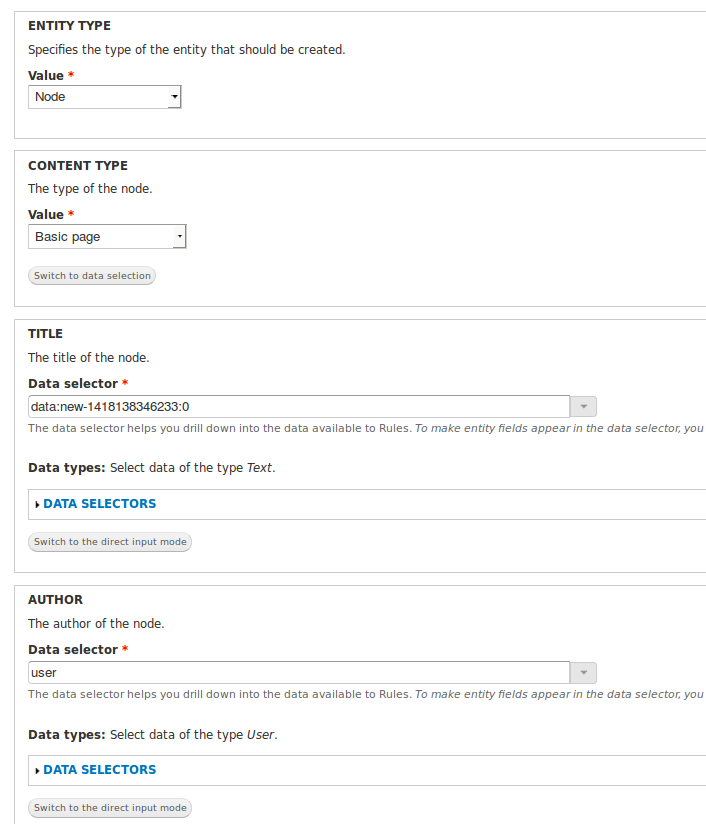This image is a screenshot of a settings pop-up menu, featuring a structured layout on a white background with black text. At the top of the menu, the heading "Entity Type" is displayed in bold black font, accompanied by the description "Specifies the type of the entity that should be created" in regular black font. 

Below this, another bold heading "Value" is present, marked with a red asterisk indicating a required field. Next to this section is a drop-down menu labeled "Node." 

Further down, another section titled "Content Type" is presented in black bold font, indicating "The type of the node." This section also includes a "Value" field marked with a red asterisk, and a drop-down menu showing "Basic page." Below this drop-down menu, a clickable gray oval button with black text reads "Switch to data selection."

Following this, there's another white box with the bold heading "Title," specifying "The title of the node." Below this, a field labeled "Data Selector" appears, also marked with a red asterisk. This section includes a drop-down menu containing the text "data:new-1418138346233:0."

The detailed layout of the settings pop-up menu highlighted here ensures that each field is clearly marked and easy to identify, providing a user-friendly interface for configuring entity and content type settings.